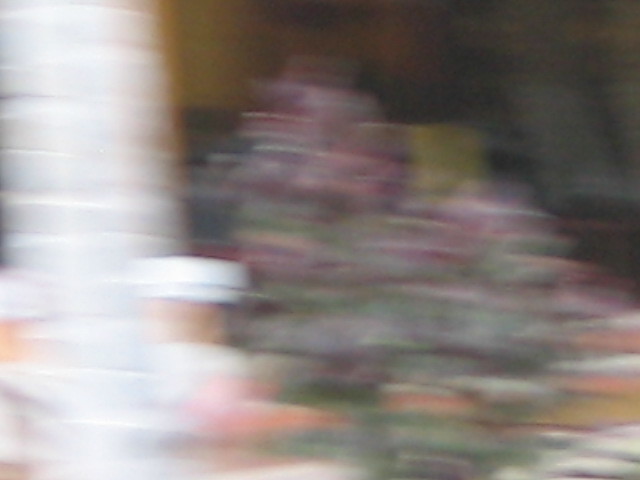A highly blurred image features what appears to be two cups of coffee, with their lids being the only somewhat defined elements. The surroundings are a mixed blur of colors, including shades of reddish-purple, green, orange, and white, suggesting the presence of trees or other vibrant objects. To the left of the coffee cups, there is a noticeable white area. In the background, a structure resembling a building is faintly visible. The photograph conveys a sense of motion or might have been affected by a camera malfunction, resulting in a distinctly distorted and abstract composition.